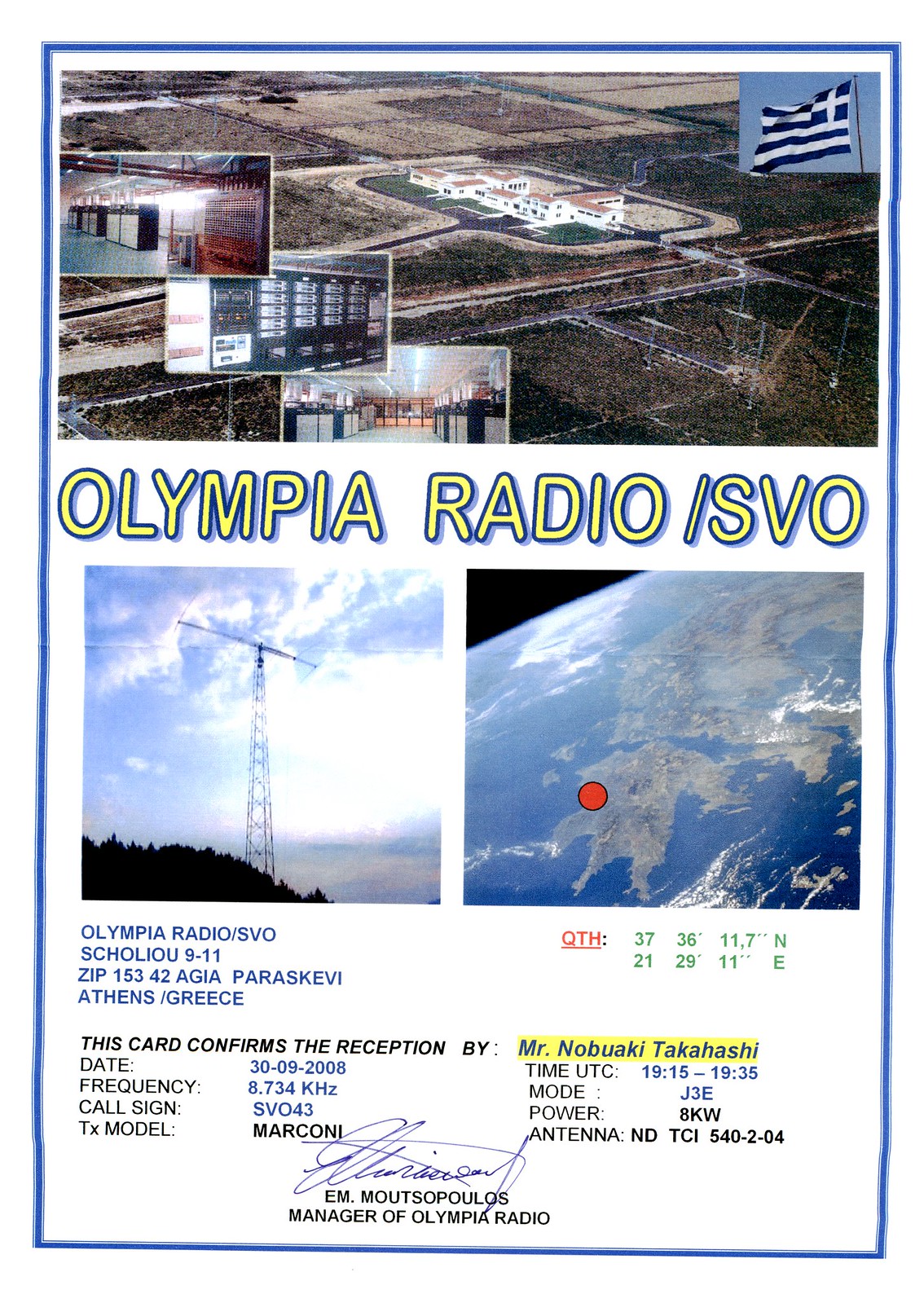The image showcases a detailed information card about Olympia Radio (SVO). The top half features a bird's-eye view of the radio broadcasting complex, comprising several low, white buildings. An inset image in the upper right corner displays a Greek flag. Overlaid on the main image are smaller photographs, likely depicting the interior of the complex, including what appears to be a computer or server room.

Below the prominent "Olympia Radio / SVO" header, there are two additional images: one of a tall broadcasting antenna and another showing Greece from space, with a red dot indicating the location of the radio station on the continent. Further down, the card provides detailed information, including coordinates (QTH: 37 36 11.7 N, 21 29 11 E), and confirms the reception by Mr. Norio Takahashi. Additional details like date, frequency, call sign, mode, power, antenna type, and other technical specifications about Olympia Radio are also listed.